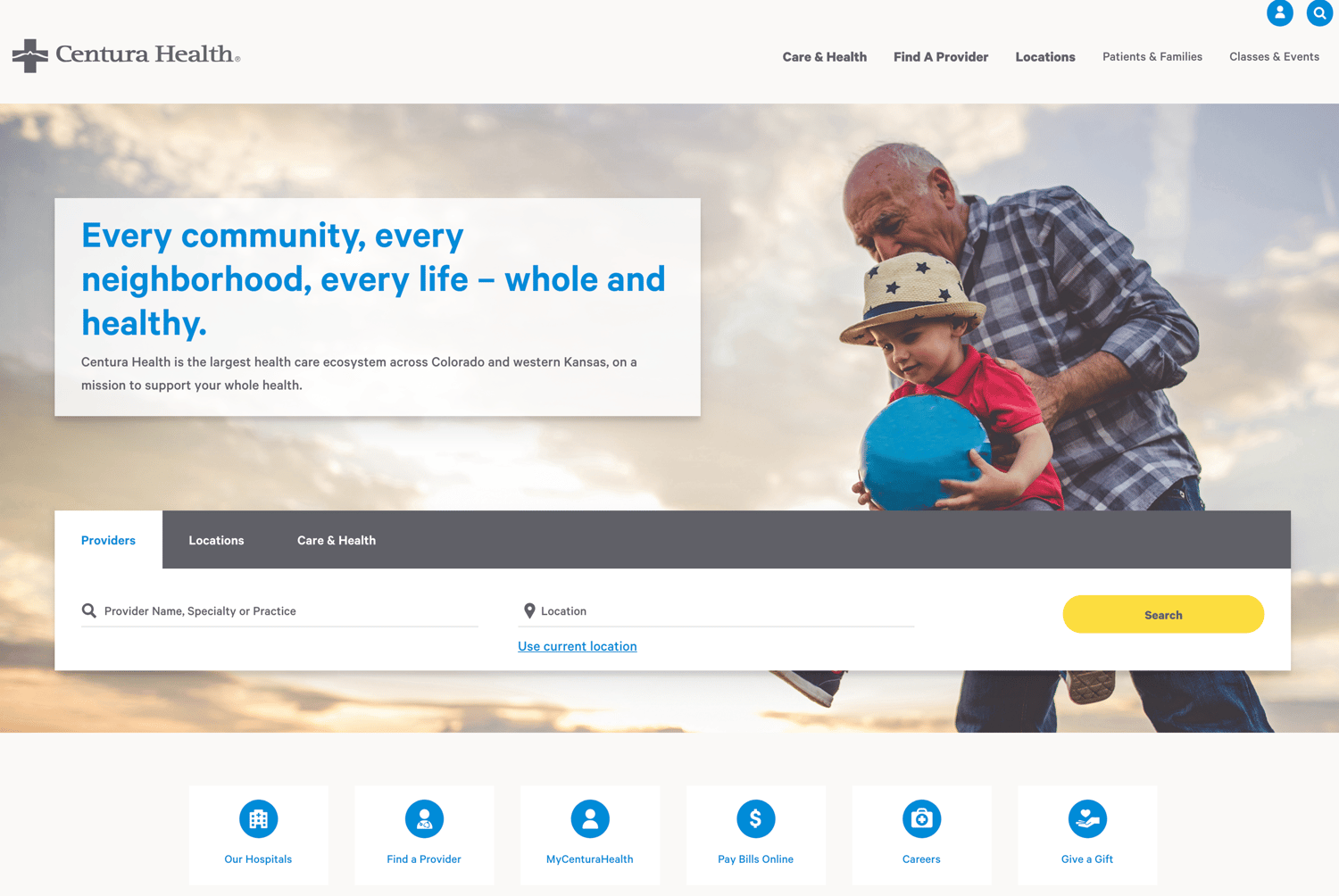Screenshot of the Centora Health homepage. The top left corner prominently displays the name "Centora Health." On the right side, several navigation tabs are visible: "Care and Health," "Find a Provider," "Locations," "Patients and Families," and "Classes and Events." Below the navigation bar, a white box features the slogan: "Every Community, Every Neighborhood, Every Life, Whole and Healthy." The text elaborates, stating that Centora Health is the largest healthcare ecosystem in Colorado and western Kansas, dedicated to promoting comprehensive health for all. At the bottom of the screenshot, a search bar allows users to enter provider names, specialties, or practices, with an option to select their current location for more accurate results.